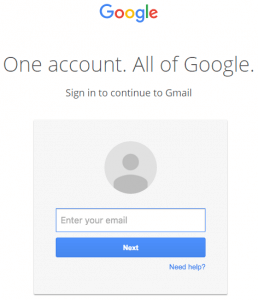The image depicts Google's sign-in page for accessing Gmail. At the top, the iconic multi-colored Google logo is prominently displayed. Below it, a message states, "One account, all of Google. Sign in to continue to Gmail."

The primary section of the page asks users to enter their email address in a designated input field. The surrounding area of the input field is a light gray, contrasting with the white background of the rest of the page. Just beneath the input field is a blue 'Next' button, which users must click to proceed to the password entry step. If the email is recognized, users will then be prompted to enter their password on the subsequent page.

Additionally, there is a 'Need help?' link located directly below the 'Next' button, offering assistance to users who may have trouble signing in. For those who have previously signed in, their profile picture may appear in a designated area on the page.

This sign-in process, which Google implemented a few years ago, differs from the traditional format where both email and password were entered on a single page. Now, by splitting them into separate pages, Google presumably enhances the security of the login process. Users typically remain signed in across various Google services, such as Google Drive, when using the same browser session.